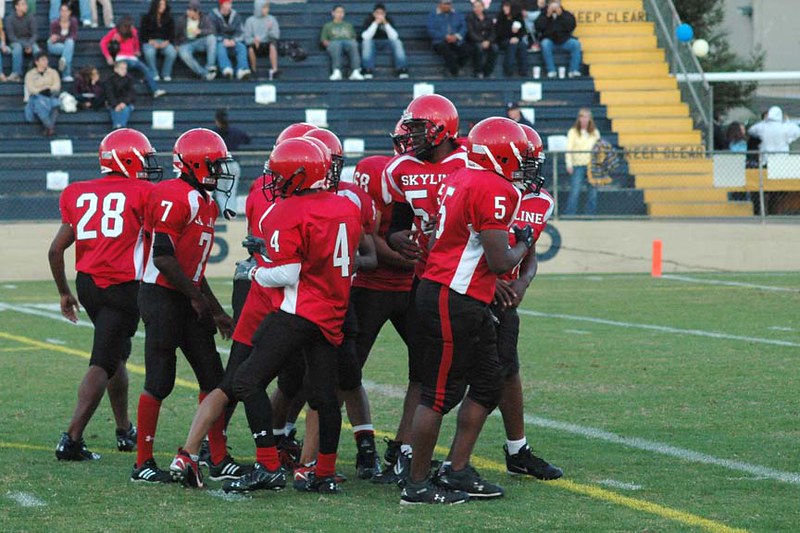The full-color photograph depicts a youth football team huddled up on a green field, preparing for their game. The team consists of around nine young black boys, all uniformly dressed in striking red football jerseys with white stripes and black pants with red stripes. The jerseys feature the team name "Skyline" prominently on the front, along with player numbers displayed on the back, front, and shoulders. They wear matching red helmets with black face guards, and black cleats from various brands. Some players sport red, white, or no socks at all.

The field itself is neatly marked with yellow and white lines and edged with orange posts to denote its boundaries. Behind a chain-link fence, a set of blue bleachers filled with spectators can be seen, with yellow steps marked "Keep Clear." To the right, trees border the field, and balloons are tied to the fence, adding to the celebratory atmosphere. The photograph captures the energy and anticipation of an outdoor football game, showcasing the team’s unity and the supportive environment surrounding them.